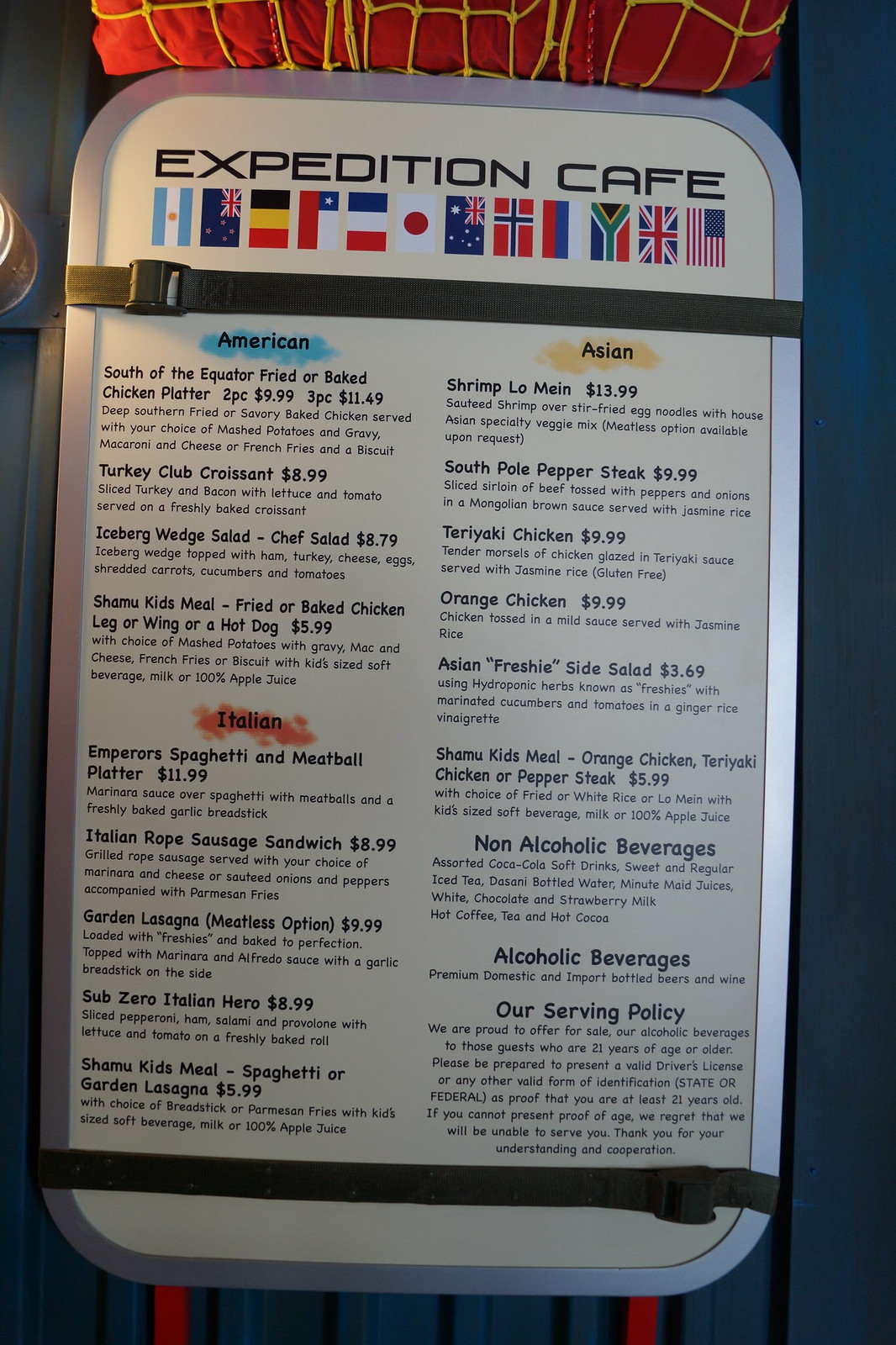The image showcases a detailed menu, affixed to a sleek metal rectangle with rounded corners. The menu is elegantly secured with leather-like bands, one at the top and one at the bottom. At the top, in bold black lettering, the words "Expedition Cafe" are prominently displayed. Directly beneath this title, there are 12 downward-facing flags representing different countries. The flag on the far right is the United States, with the United Kingdom's flag immediately to its left, and Japan's flag appearing as the fifth from the left.

The menu's layout is organized into several categories, each highlighted in distinct colors for easy navigation. The first column features the "American" section, highlighted in light blue and printed in black. This category lists four dishes, each with a bold title and a detailed description in smaller print beneath. Next, highlighted in red, is the "Italian" section, which offers five different dishes.

Continuing to the next column on the right, the "Asian" section is highlighted in yellow and also contains five offerings. Beneath this section, a series of informational categories are listed, including "Non-Alcoholic Beverages," "Alcoholic Beverages," and the cafe's "Serving Policy." The meticulous arrangement and vivid highlights make the menu both visually appealing and easy to read.